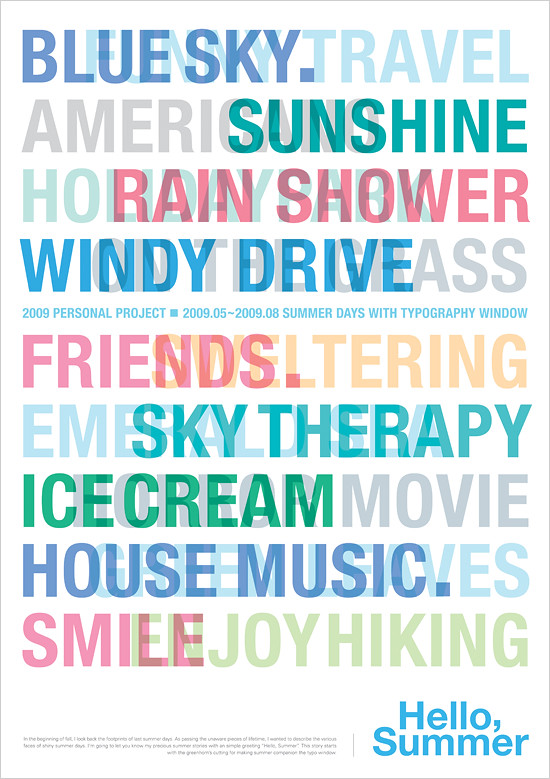The image is a vertically aligned rectangular poster with a white background and a thin gray border, filled with vibrant, overlapping typography arranged in a somewhat jumbled pattern. The poster prominently features the following text:

- At the top left, in dark blue all-caps letters: "BLUE SKY." 
- Just below "BLUE SKY," in varying colors and less solid fonts: "TRAVEL" (light blue), "AMERICANO" (gray), and "SUNSHINE" (turquoise).
- Continuing downward, phrases including "A MERRY SUNSHINE" (gray and turquoise), "A RAIN SHOWER" (red), "WINDY DRIVE" (blue), and "2009 PERSONAL PROJECT" (light blue).
- Additional overlapping words throughout the poster include "HOUSE MUSIC," "FRIENDS," "SKY THERAPY," "ICE CREAM," "MOVIE," "SMILE," "JOY," "HIKING," "HOLIDAY," and "EMERALDS," among others.
- At the very bottom right corner, in blue text: "HELLO, SUMMER."

Some smaller text near the bottom references "2009.05-2009.08, SUMMER DAYS WITH A TYPOGRAPHY WINDOW." The overall effect is a colorful, lively collage of summer-related terms, conveying a fun and vibrant seasonal vibe.